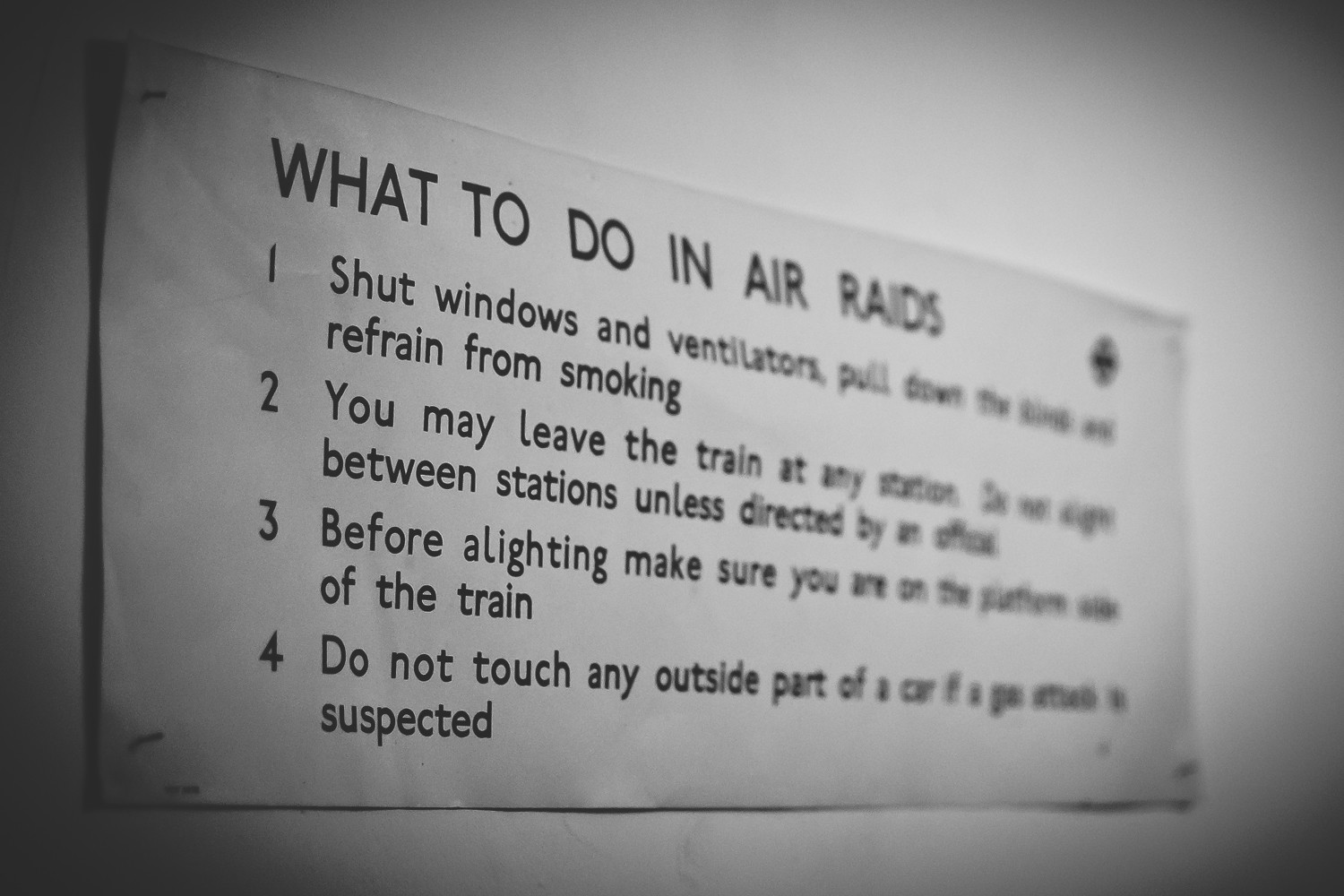This black and white photograph shows a warning plaque, possibly from the WWII era, detailing instructions on what to do during air raids. The plaque, appearing as either a scanned image or a photograph of a paper sign, is stapled or tacked onto a mostly gray background with black corners. The sign has clear black print on a white background.

The instructions are numbered one through four. 

1. **Shut windows and ventilation,** followed by a blurry section, then clearly stating, **refrain from smoking.**
2. **You may leave the train at any station,** with some blurred text, **unless directed by an officer.**
3. **Before alighting, make sure you are on the platform end of the train.**
4. **Do not touch any outside part of a car if a gas attack is suspected.**

The right side of the sign is somewhat blurred, but the main points remain legible, offering detailed guidance for safety during air raids.